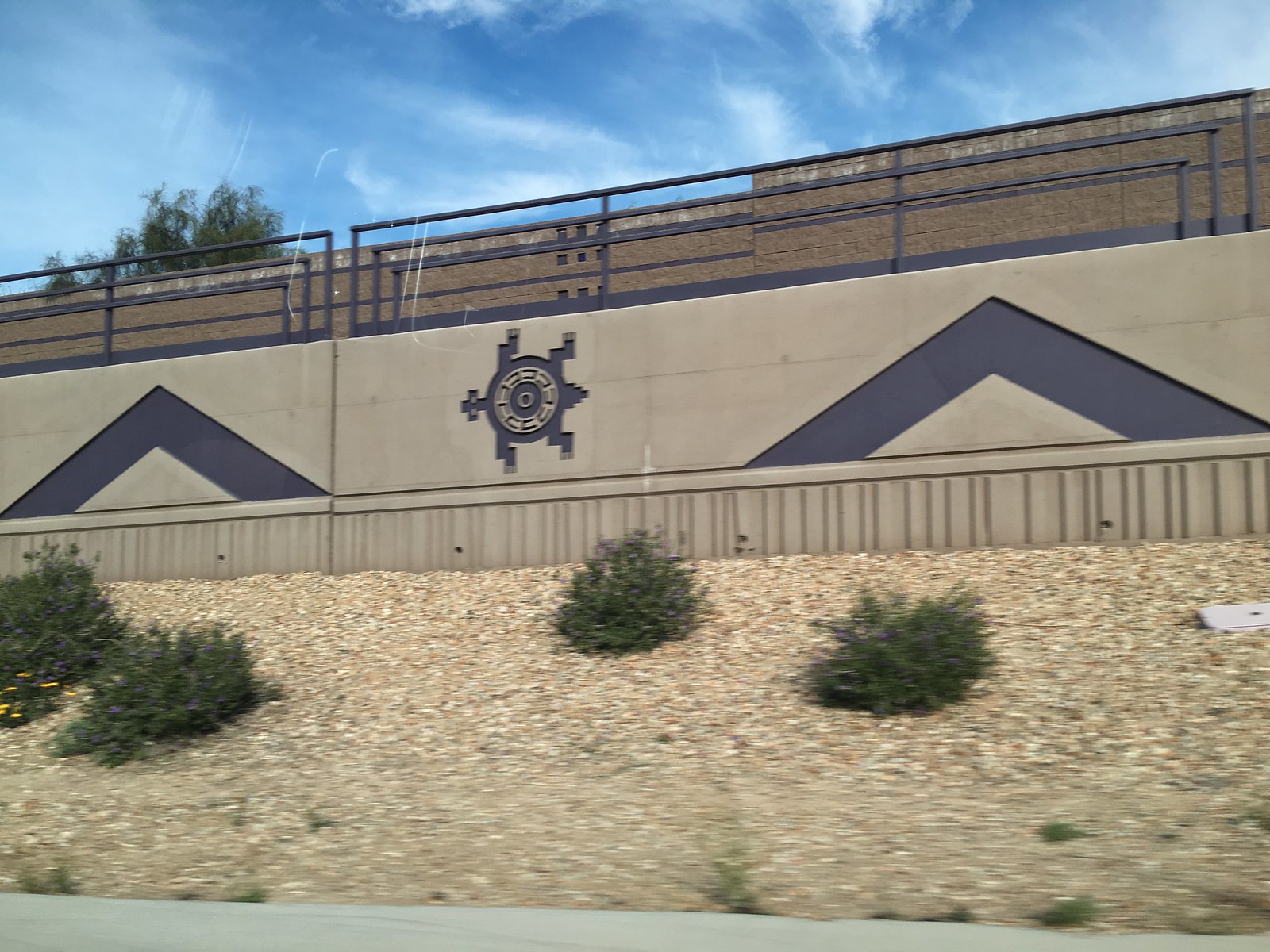A photograph taken from the window of a moving vehicle on a freeway captures a vibrant scene against a backdrop of a clear blue sky adorned with wispy cirrus and mare's tail clouds. The frame looks upward along an incline blanketed with small tan gravel and scattered with a few green bushes. Central to the image is a tan-colored wall featuring a striking Native American design. A stylized geometric turtle takes prominence, flanked symmetrically by the tops of two dark triangular bands. Above these elements, metal bars, painted to match the turtle and triangles, extend horizontally. Rising behind this decorative wall is a structure that appears to be constructed from brick, adding depth to the composition. The upper edges of this structure give way to the expansive sky, accompanied by a glimpse of treetops peeking from behind.